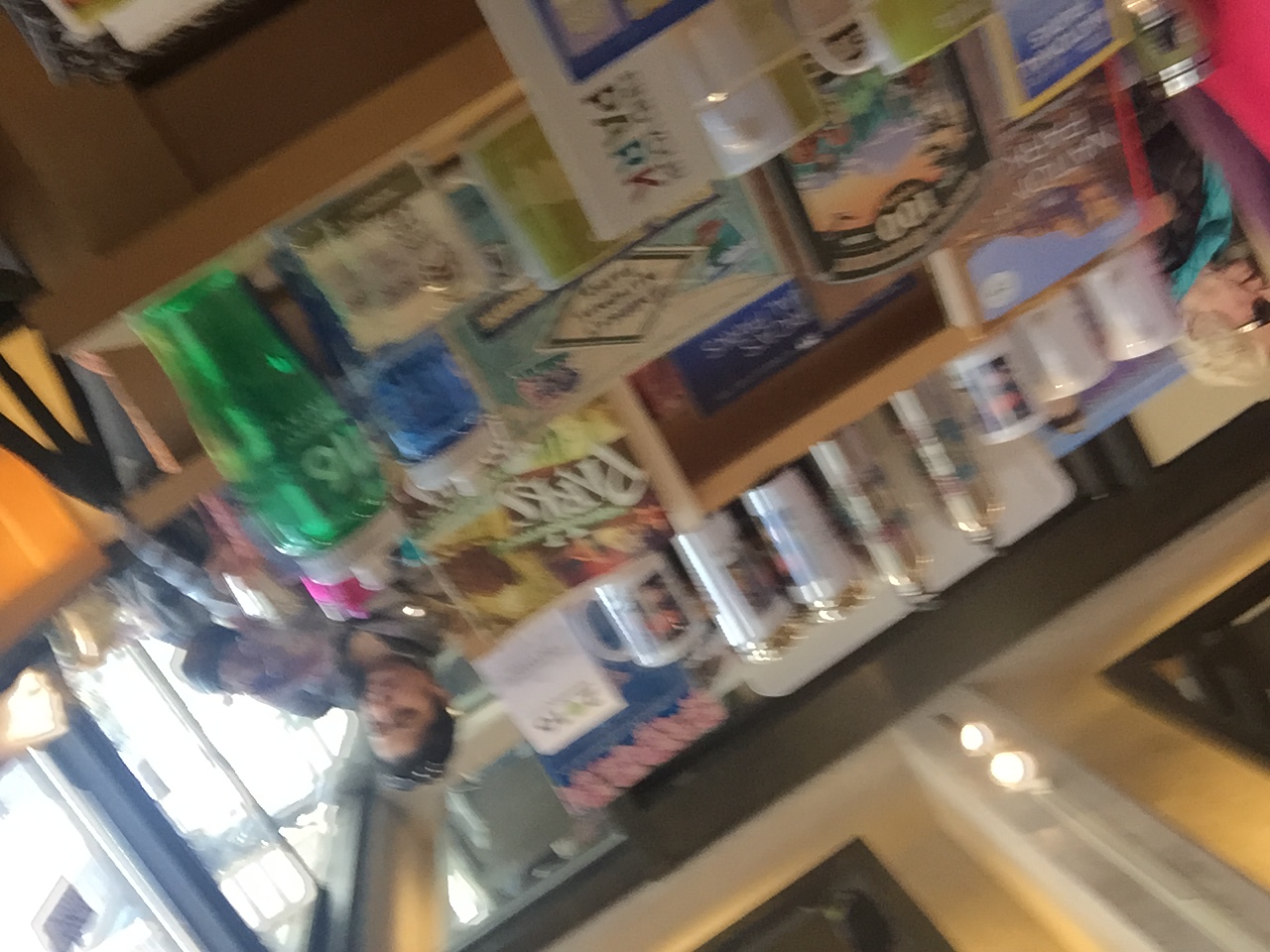In a brightly lit store, shelves brimming with a variety of products are neatly organized. The top shelf displays an assortment of cups, some adorned with park-themed designs. Below, a variety of cans and spray bottles are visible, alongside more cups, suggesting a focus on outdoor or park-related merchandise. Partially obscured by the edge of the frame is a product with the word "park" faintly visible, adding to the thematic coherence of the display.

The store’s environment is well-illuminated by overhead ceiling lights, which highlight the organized chaos of the retail space. Two women are present in the image. One appears to be an older white lady with white hair and glasses, presumably browsing the items. Nearby, a woman who looks Spanish, with dark hair and sunglasses resting on her head, is engrossed in her phone. This scenario captures a moment of everyday life within the context of a store celebrating parks and outdoor enjoyment.